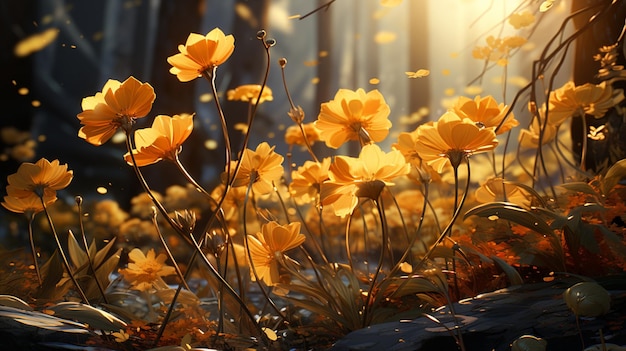This beautifully detailed image, which has an almost animated quality, captures a vivid portrait of a bed of yellow and golden flowers resembling sunflowers. These flowers, with their many petals and skinny stems, appear to be blooming and reaching up towards the sky. They are clustered together, creating a dense and interconnected field. The vantage point of the image is as if looking up through the flowers, emphasizing their height and vibrancy. In the background, you can see a dense forest with dark tree trunks, adding a sense of depth. On the right side, sunlight peeks through the trees, casting a warm light that reflects off the flowers. Amidst the flowers, on the bottom right, there is a solitary dark rock surrounded by green and red leaves, and on the left side, another small dark blue rock is visible. Behind the flowers, towards the bottom, there's a small pond, adding a serene touch to the forest scene. The overall lighting creates a mix of bright highlights and shaded areas, enhancing the natural beauty of the setting.